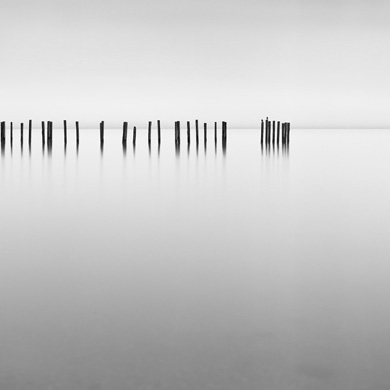The image is a square-shaped photograph or digital art piece with subtly differing height and width proportions. Dominated by shades of gray and white, the scene evokes a tranquil and still atmosphere. The horizon line, about one-third down from the top, delineates a smooth transition from the light gray sky to the barely rippling, reflective water below. Emanating from the left side are a series of thin, black, vertical lines or poles, which could be remnants of a wooden pier or bridge. These poles gradually fade at their bases, creating an impression of submersion or reflection in the calm, flat waters. The overall ambiance is serene, and the subtle details, including the thin, varying shapes of the poles and their ghost-like reflections, enhance the composition's ethereal quality.